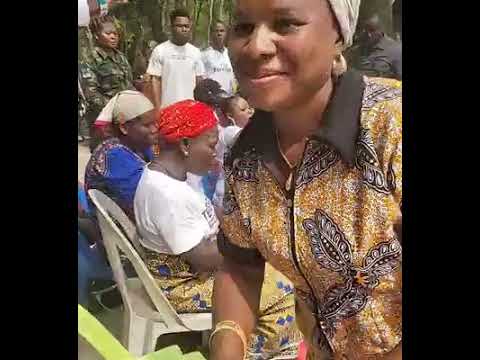The image depicts a group of African or African-American individuals, focusing on a woman in the foreground who appears to be taking a selfie. She is wearing a yellow and brown floral patterned shirt with a brown collar and zipper front. She has hoop earrings, a gold bracelet, and a white head wrap. Her right arm is visible, suggesting she is using her left arm to hold the camera. The background features a mix of four or five seated and three or four standing individuals, some in traditional African clothing and others in plain outfits like white t-shirts. Notably, a seated woman wears a red head wrap with a white t-shirt, while another has a white head wrap and a blue t-shirt. The overall scene suggests a communal event, with everyone appearing joyful and engaged. The photo is grainy, potentially due to motion or low-quality capture, and is framed with black columns on either side.